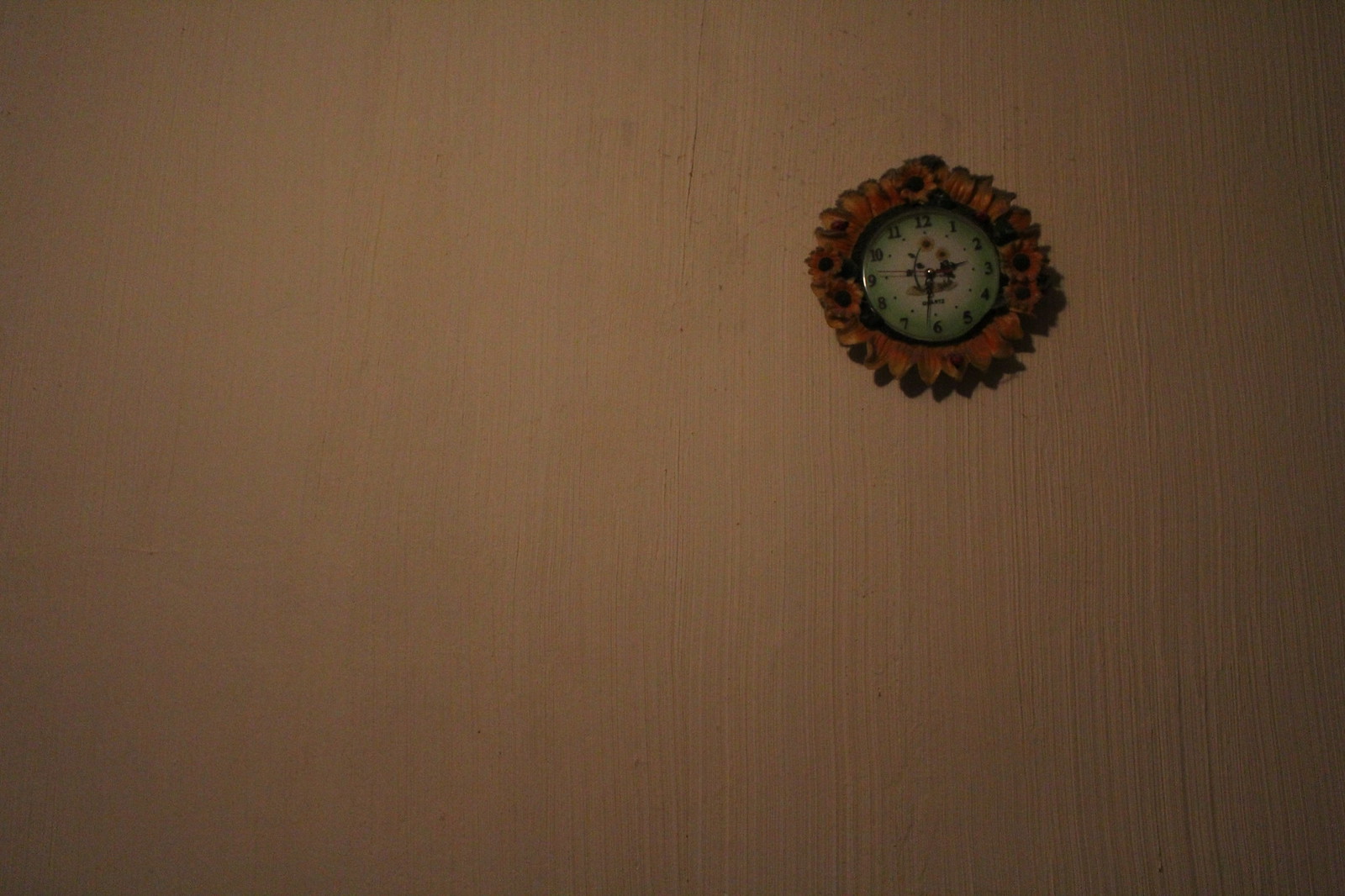The image captures a small, sunflower-shaped wall clock positioned slightly right of center and about two inches from the top on a peachish white wall. The wall itself has a textured appearance, suggesting it may be poorly painted or wallpapered with a wood grain pattern. The clock is composed of brown petal-like protrusions encircling the frame, transitioning from a greenish hue at the outer edge to a white gradient in the center. Black numbers encircle the clock face, which features two black hands and a thin red second hand. In the very center, two small sunflower illustrations add a decorative touch. The lower left side of the clock casts a subtle shadow on the wall, enhancing the slightly dark and underexposed atmosphere of the room and contributing to its somewhat eerie, sinister vibe.